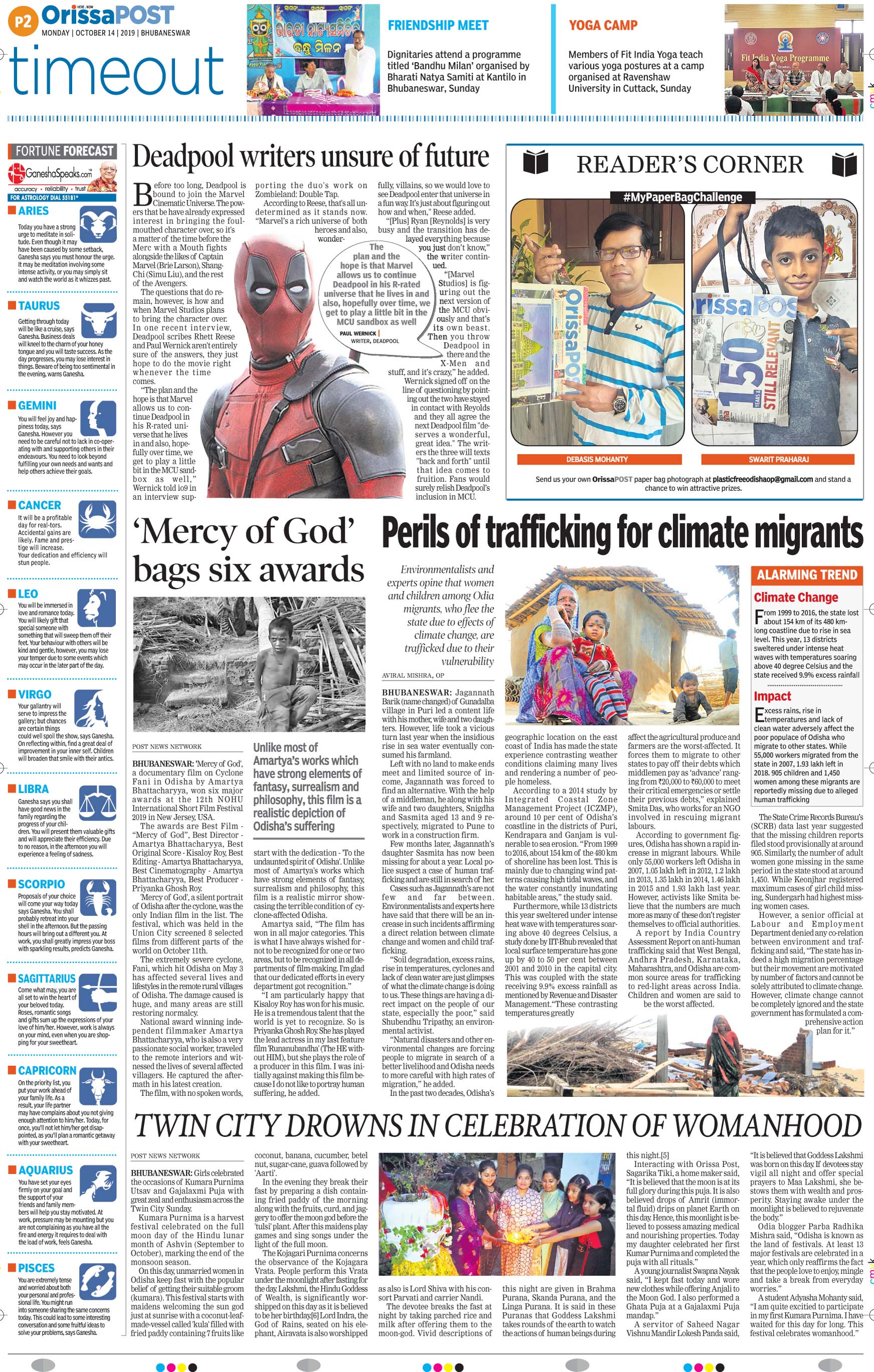The image depicts the front page of the "LRISSA Post," dated Monday, October 14th, 2019, printed in Bhubaneswar. The main headline reads, "Deadpool Writers Unsure of Future," accompanied by several other intriguing headlines including, "Mercy of God Bags Six Awards," "Perils of Trafficking for Climate Migrants," and "Twin City Drowns in Celebration of Womanhood."

On the far left of the newspaper, a fortune forecast section showcases predictions for all zodiac signs. The top feature in this section highlights a significant event, titled "Friendship Meet," which includes dignitaries attending a program known as "Bandhu Milan," though specifics are sparse due to the complex Indian names. Additional sections include a Yoga Camp, Reader's Corner, and an interactive "My Page, My Paper Bag Challenge," which displays creative items made from newspaper.

The page is vibrant with a palette of colors including white, blue, pink, orange, red, yellow, green, and purple, enhancing the visual appeal and drawing the reader's attention to various points of interest.